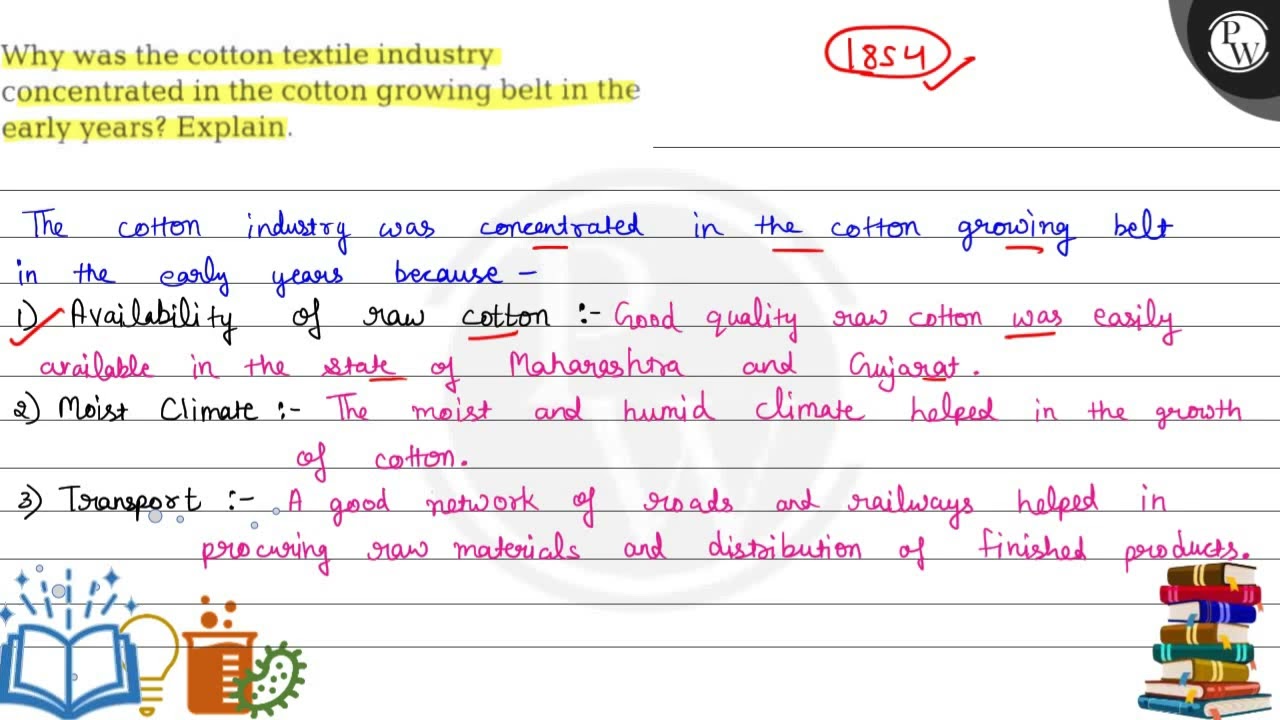This image is a landscape-oriented index card filled with notes and various elements. At the top, centered in black text and highlighted in yellow, is the question, "Why was the cotton textile industry concentrated in the cotton growing belt in the early years?" Beside this, the number "1854" is prominently handwritten within a red circle with a checkmark. Below the question, in blue ink, the explanation begins: "The cotton industry was concentrated in the cotton growing belt in the early years because..." followed by three detailed points. Pink and black text provide additional elaboration, noting the availability of high-quality raw cotton, specifically from the state of Gujarat. Towards the bottom, on the left, there are colorful printed images, including a blue book, a yellow lightbulb, a red bubbling beaker, and a green worm. To the bottom right, there is a stacked array of books in various colors. Additionally, in the upper right-hand corner, a black logo with the letters "PW2" is visible.